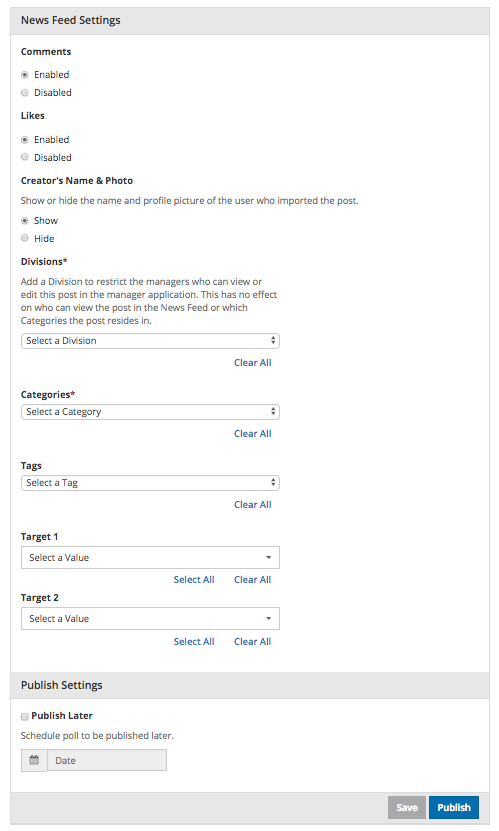The screenshot titled "News Feed Settings" features a structured interface for managing the visibility and organization of posts within the application. 

At the upper left-hand corner, "News Feed Settings" is prominently displayed in black text on a gray bar. Below this, a well-organized list allows users to control various aspects of their news feed.

1. **Comments:**
   - Shown in black font.
   - Enabled option is checked; Disabled option is shown in lighter gray font below.

2. **Likes:**
   - Displayed in dark black font.
   - Enabled option is selected; Disabled option in gray.

3. **Creator’s Name and Photo:**
   - "Creator's name and photo" in darker black font.
   - Description in gray font: "Show or hide the name and profile picture of the user who imported the post." 
   - Option to Show is checked, with Hide as an alternative.

4. **Divisions (marked with a red star):**
   - Detailed instructions: "Add a division to restrict the managers who can view or edit this post in the manager application. This has no effect on who can view the post in the news feed or which categories the post resides in."
   - A selection bar with "Selected division."
   - "Clear all" in blue text beneath on the right.

5. **Categories (marked with a red star):**
   - A selection box labeled "Select a category."
   - "Clear all" in blue at the bottom right.

6. **Tags:**
   - "Tags" in black font.
   - A search box labeled "Select a tag."
   - "Clear all" in blue on the lower right.

7. **Target One and Two:**
   - Each in black font with their own search box marked "Select a value."
   - Options for "Select all" and "Clear all" in blue text on the lower right of each box.

At the bottom is a gray bar labeled "Publish Settings" in black. 

8. **Publish Settings:**
   - "Publish later" option with an unchecked box.
   - Instruction in gray: "Schedule post to be published later."
   - A calendar icon with a gray box labeled "Date" for date selection.

Finally, at the bottommost gray banner:
- The "Save" button is grayed out with white font.
- The "Publish" button is blue with white font, ready for user interaction.